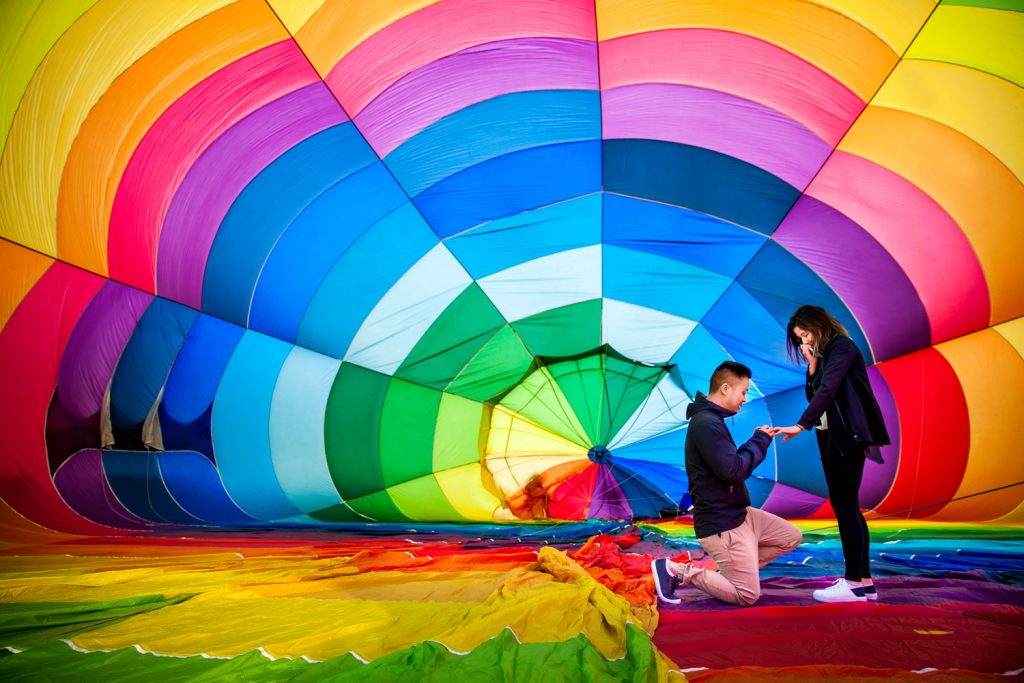In this intricately staged photograph of a marriage proposal, a young couple, likely in their mid-20s and of Asian descent, occupies the right-hand portion of the image. The man, dressed casually in a dark hoodie, khaki pants, and blue sneakers, is down on one knee, proposing to the woman. He is placing a ring on her outstretched right hand while she stands slightly to his right, visibly moved with her left hand held up to her face in astonishment. The woman is clad in a black top, black pants, and white sneakers with pink accents.

The photograph's composition features a vibrant and structured background, accentuated by the fabric of what appears to be an inflated parachute or hot air balloon. This multicolored fabric covers both the ground they stand on and the backdrop, creating an eye-catching, rainbow-hued setting. The fabric starts in a dark blue at the center and fans out in a circular pattern with stripes of green, purple, pink, orange, and yellow, among other colors, lending a whimsical and celebratory atmosphere to the scene. The parachute or balloon material, likely made of silk or nylon, is held aloft behind them, suggesting the presence of a wind machine or other means of inflation, adding to the carefully crafted and striking visual appeal of this joyous moment.